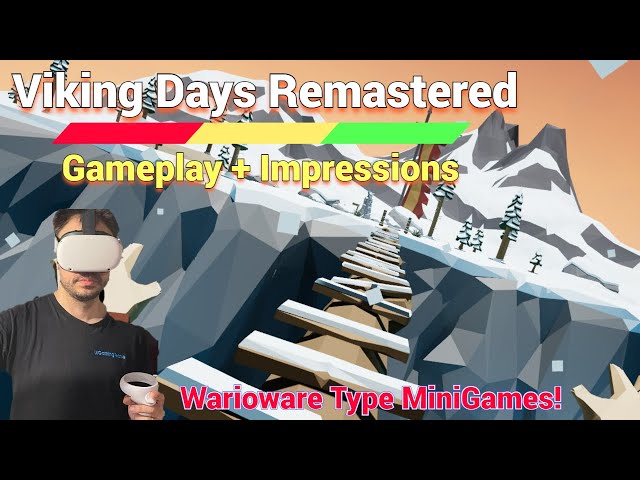The image is a rectangular video thumbnail for a VR video game, with thick black borders on the top and bottom. In the center of the image, white text at the top reads "Viking Days Remastered," followed by yellow text that says "Gameplay Plus Impressions." At the bottom, there's red text with a white border stating "WarioWare Type Minigames!" In the bottom left corner, a man wearing a VR headset, which is white on the front and black around his face, holds a round white controller. He is dressed in a black shirt with a blue logo. The background of the image, which appears to be an animated drawing, depicts a snowy landscape featuring a bridge over a chasm, large gray mountains with white snow, and evergreen trees also covered with snow. This likely represents the game's setting seen by the VR player.